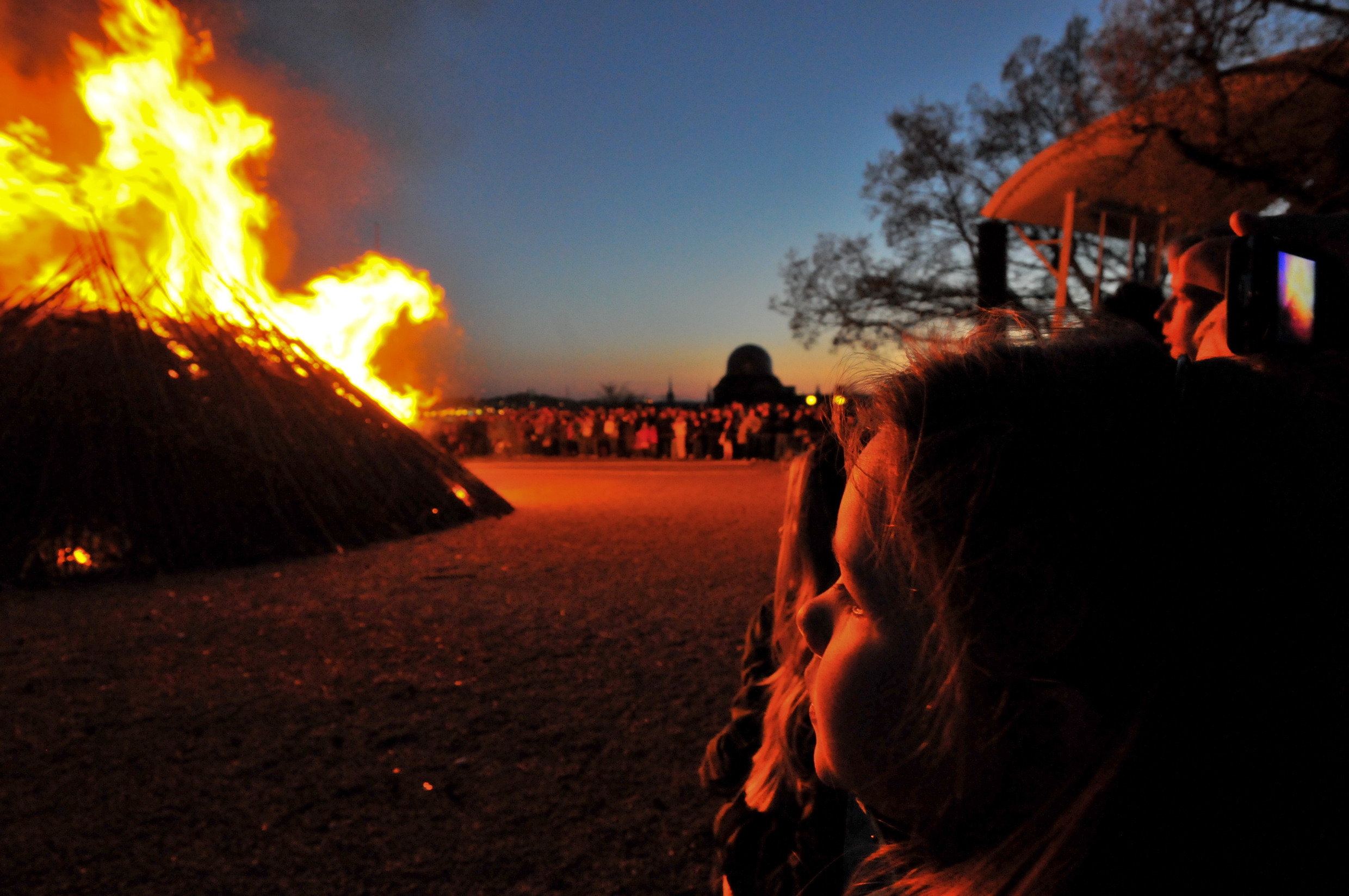The photograph captures a dramatic scene at night, likely taken at a festival such as Burning Man. Dominating the left side is a towering bonfire, roughly 10 feet tall, shaped like a cone or teepee, roaring with vibrant flames in hues of yellow, orange, and red. The sky above transitions from deep, dark blue to shades of purple and hints of sunset orange.

In the foreground, a young girl, positioned on the right side of the image, gazes intently at the fire. Her profile is illuminated by the bonfire's glow, casting an orange-red reflection on her face, creating a striking contrast against the surrounding darkness. Behind her, partially obscured, are other people, including an older woman, also absorbed by the spectacle.

The crowd, numbering in the hundreds, forms a large, distant circle around the fire. The photo has a dim, almost mysterious quality, with the faces of the distant onlookers barely discernible, except for the red and orange highlights from the flames. On the far horizon, a building with a domed top is faintly visible, and some sparse trees and a small canopy are dotted around the background. The ground appears dark but reflects the fire's intense color, casting a reddish tint over the scene. The overall mood is a mix of awe and quiet observation, capturing a communal moment of fascination with the blazing bonfire.